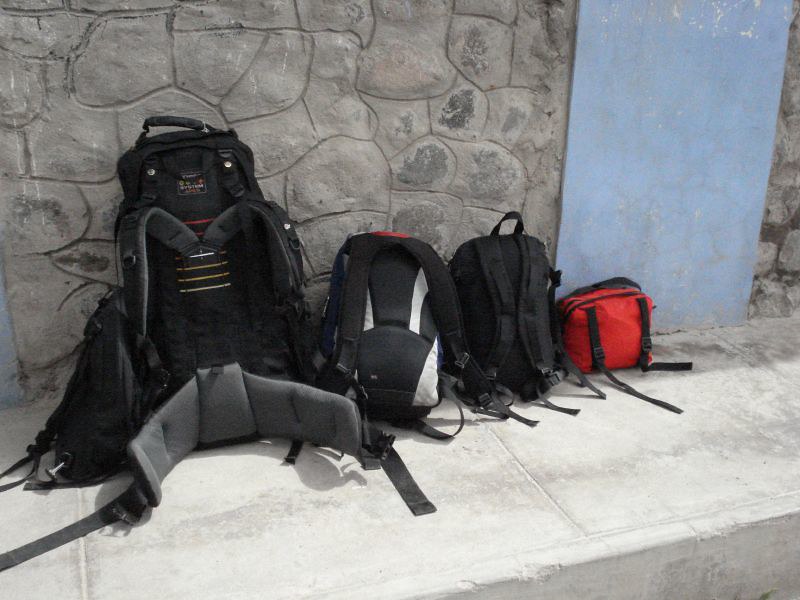This detailed color photograph showcases four diverse backpacks arranged in a row on a light gray diagonal cement sidewalk that extends from the bottom left to the lower right-hand side of the image. The backpacks rest neatly against a gray stone wall with large, irregularly sized stones and dark gray grout. Starting from the left, the largest backpack is black with a padded waist belt, silver adornments, white lines, and a sturdy top handle, making it suitable for hiking or traveling. Adjacent to this is a smaller black backpack with grey highlights and a distinctive red handle. The third in line is a solid black backpack, sleek in design. At the far right is a small, bright red canvas carry-on bag with black handles and webbing, adding a pop of color to the scene. The gray rectangular shape nearby suggests the presence of a door. The sidewalk's clean appearance and tall curb further detail this urban setting.